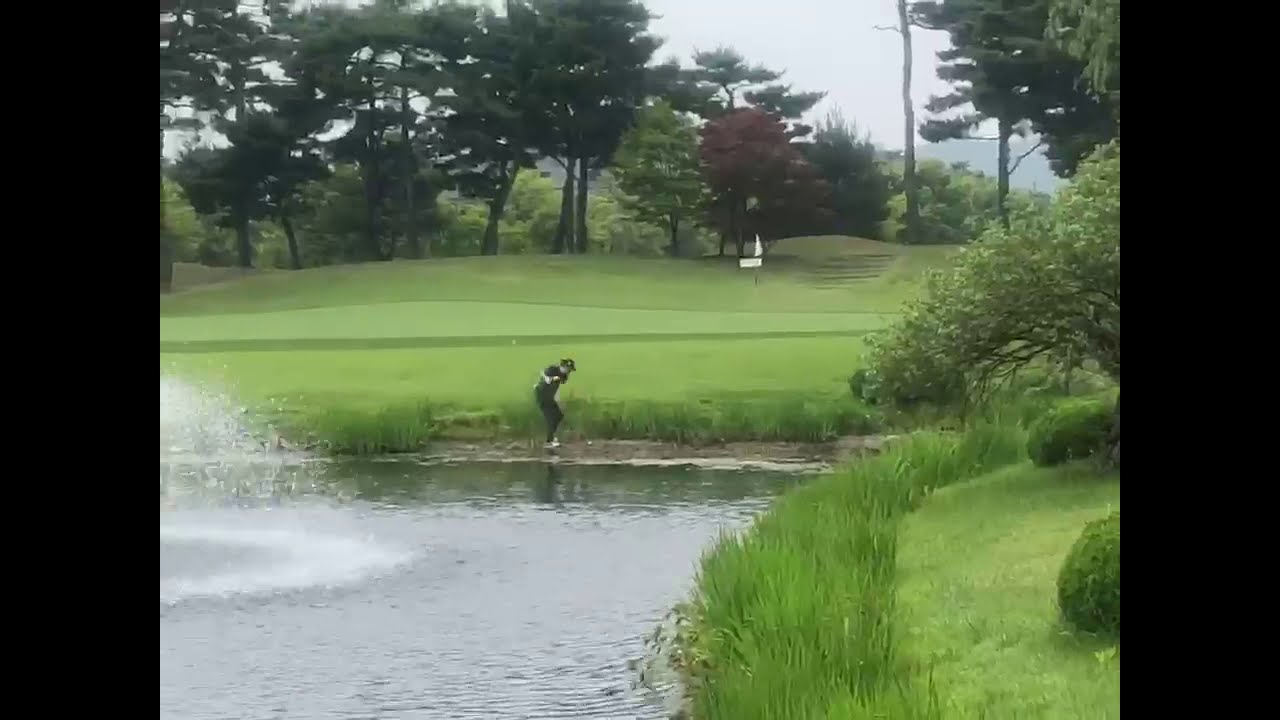The photograph captures a golfer on a well-maintained golf course, taken on a bright but cloudy day. The individual, dressed in black attire and a matching cap, is shown in mid-swing at the edge of a water trap, with their knees bent and arm raised, aiming to hit a tiny white golf ball. The scene features a small pond in the lower left corner, complete with a cropped fountain spewing water. Tall grass surrounds the water trap, adding to the challenge. The lush green fairway extends towards a white flag planted further up a hill. The background is adorned with large trees and some bushes to the right of the water. The image is framed by tall black bars running vertically down each side, and the entire setting is naturally lit, indicating it is daytime.